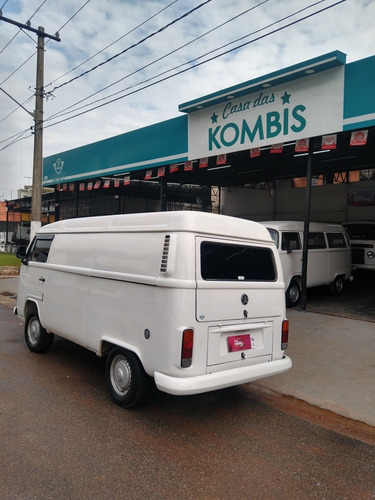The image depicts the front of a shop named "Casa das Kombis," a business likely dealing in vintage VW vans. The building has a teal-colored facade with a white rectangular sign displaying the name "Casa das Kombis" in turquoise letters, flanked by two green stars. The structure features an open-air carport, supported by black poles, underneath which an old-school white van and a moving truck are parked. A similarly styled white van, recognizable by its Scooby-Doo-like wheels and pink license plate, is parked on the street in front of the shop. The shop is adorned with red banners hanging from the edge of the roof. To the left of the scene, an electric pole stands with power and telecommunication lines running from it. The background displays a daylight sky filled with numerous clouds.